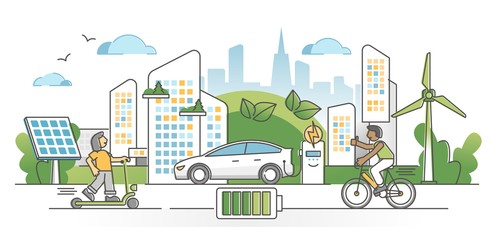The image is a hand-drawn, cartoonish scene set against a solid white background, emphasizing an eco-friendly environment. In the center of the scene is a whitish-gray Prius-like vehicle with blue windows and black wheels, positioned near an electric charging station distinguished by a yellow lightning bolt sign above it. The road the car is on is outlined in black and white, leading towards the nine o'clock position.

Adjacent to the car, there's a young black boy wearing a green sleeveless shirt and white pants, riding a yellow bike to the left. On the opposite side, a Caucasian girl with long, dark gray hair, dressed in an orange shirt and blue pants, rides a green scooter with small black wheels and a headlamp, heading towards the three o'clock position.

Central to the scene is an image of a battery with five green bars, symbolizing sustainable energy. The backdrop features tall, white city skyscrapers with blue, yellow, and dark blue windows, a blue solar panel grid on the left, a green windmill on the right, and a green hill adorned with foliage. The sky above includes blue clouds and birds, enhancing the depiction of a clean, eco-friendly urban environment.